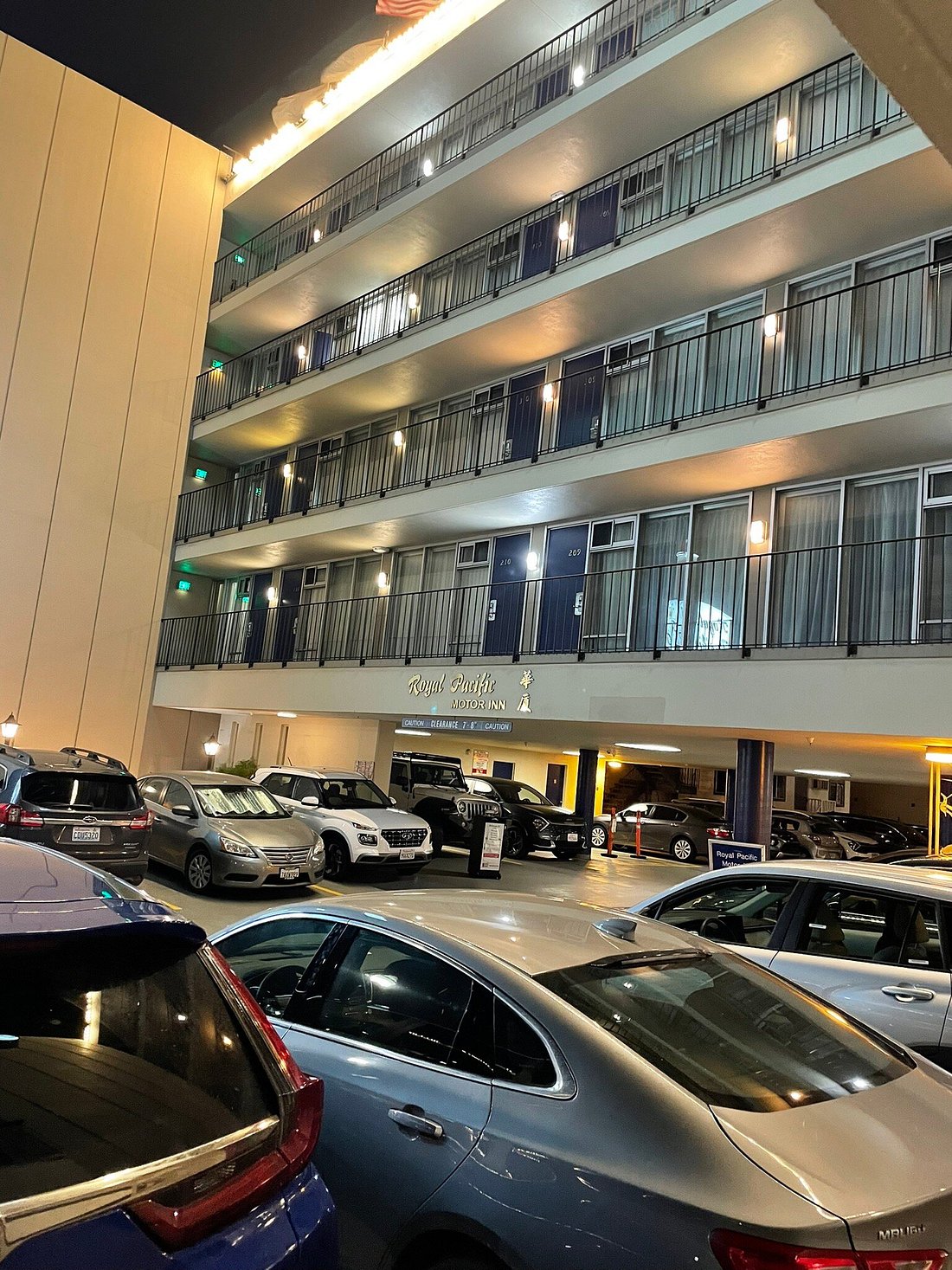This detailed photograph captures the Royal Pacific Motor Inn, a four-story establishment located in what appears to be a bustling metropolitan area. Dominating the upper section of the image is the hotel itself, characterized by its grayish-white facade and identifiable signage. Each room features three person-height windows adorned with drawn curtains, possibly glass doors leading to balconies secured by black metal railings. Blue doors, illuminated at night by overhead lights, line outdoor walkways on each level.

The first floor transitions into a parking garage, supported by pillars that extend up and support the structure, while additional parking is visible in front of the building. This ground-level garage and outdoor lot host a variety of cars and SUVs. The lower portion of the image focuses on the parked vehicles, set against the backdrop of illuminated rooms and the industrial-style architecture of the hotel.